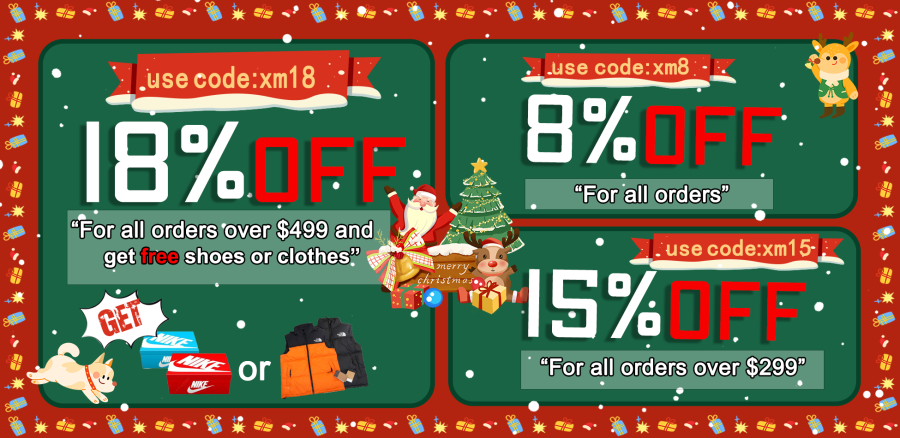The image depicts a festive coupon-themed website advertisement. The background is a bright red rectangular frame adorned with a lively border featuring a variety of holiday designs including wrapped presents, gift bags, stars, and Santa hats. These decorations are in an array of vibrant colors like yellow, red, and blue, giving the whole image a cheerful holiday atmosphere.

Prominently displayed within this festive border are three coupons, each offering different discounts. On the left side, occupying nearly half of the space, is an 18% off coupon applicable to all orders over $499. This coupon also includes a promotion for free shoes or clothing with the purchase, showcasing visuals of two Nike shoe boxes and two vests. The details for this offer are highlighted with a mix of white, red, black, and a touch of green fonts, and the specific code to use is "XM18".

To the right of this large coupon, there are two smaller offers. One provides an 8% discount on all orders, while the other gives a 15% discount for orders over $299. The text for these coupons is similarly styled with a festive and easy-to-read font. The overall design is engaging and visually appealing, perfectly capturing the holiday spirit while encouraging purchases.